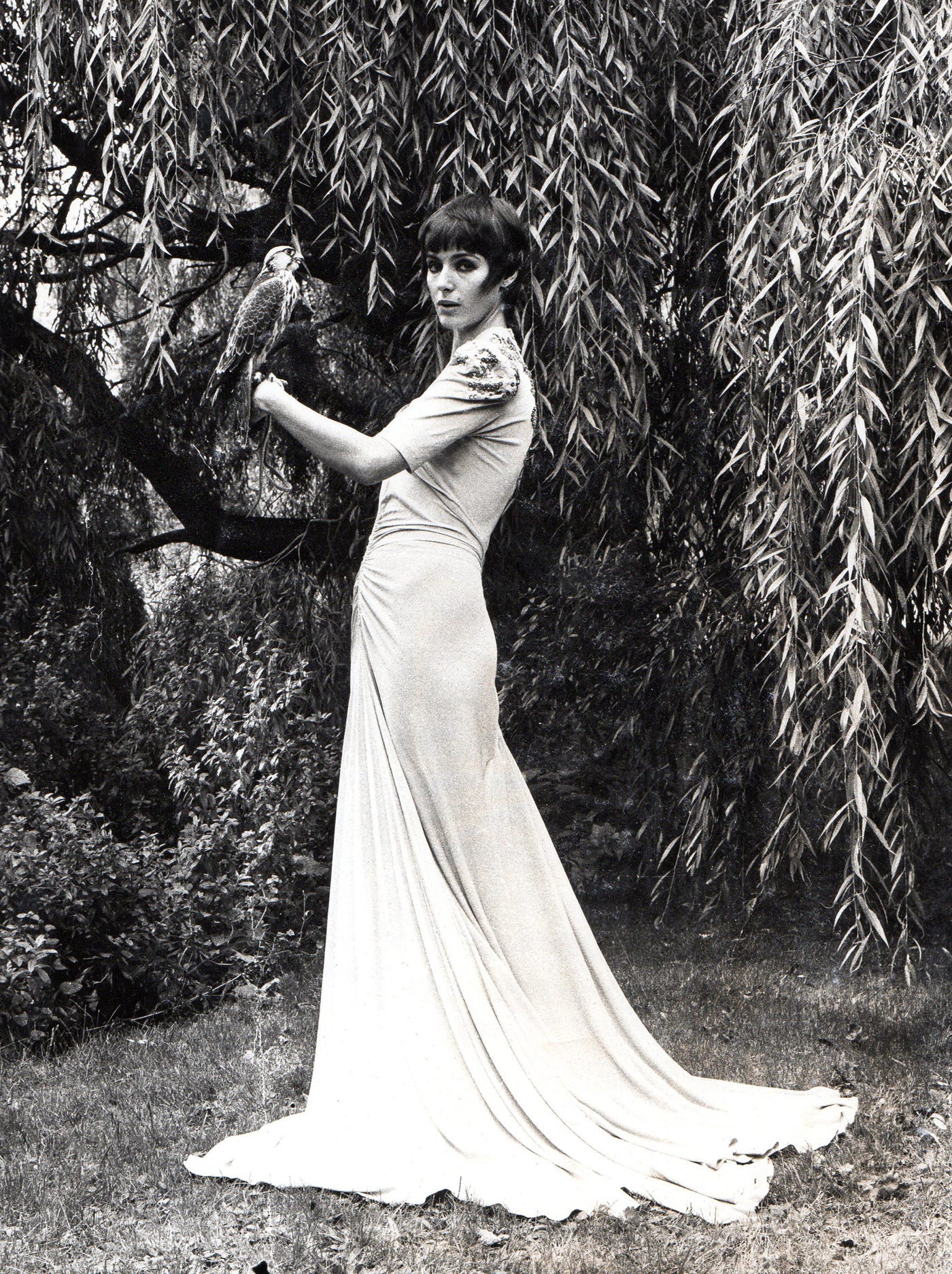In this black and white photograph, a slender woman is elegantly posed in front of a sprawling weeping willow tree, whose long branches with numerous small leaves flow downwards. She stands on a well-kept lawn, adorned with scattered dried leaves and surrounded by dense bushes and hedges. The woman's short, dark hair, styled just above her eyes and over her ears, frames her face and features prominent sideburns along her cheekbones. She has a mole on the left side of her lip and wears dark eye makeup, giving her a somewhat intense, blank stare, with her mouth slightly open.

She is dressed in an exquisite, flowing white gown that drapes elegantly to the ground, extending about 30 centimeters around her feet. The dress has a intricate floral or lace design on the shoulders and falls to sleeves that extend most of the way to her elbows. In her left hand, she holds a bird, possibly a parrot or falcon, perched gracefully on her index finger. The bird's gray feathers blend harmoniously with the grayscale background of the weeping willow, creating a seamless and hauntingly beautiful scene. The overall composition, reminiscent of an elegant wedding photo, captures a moment of serene beauty amidst the natural surroundings.